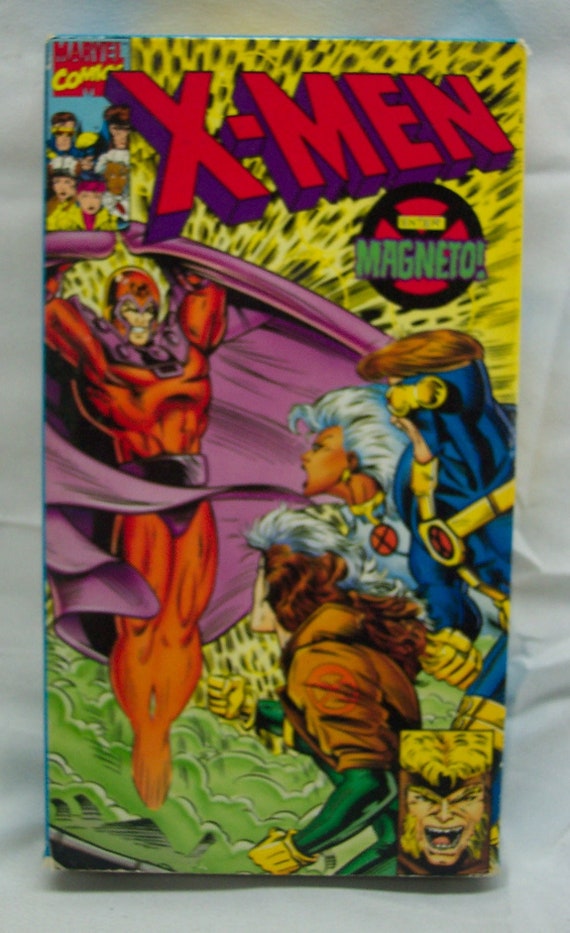The image features a portrait-oriented photograph of a comic book cover with a textured, light-colored, wrinkled background. The comic book is titled "X-Men," prominently displayed in large red text with a purple shadow at the top. The background of the title area is yellow with black leopard-print-like lines. Below the title, a black circle with red inside is crossed with black lines, bearing the green text "Magneto!" accompanied by an exclamation mark.

In the top left corner, the text "Marvel Comics" is present alongside a picture of cartoon characters. Dominating the cover is Magneto, depicted wearing a red skintight suit with a swirling purple cape, extending from his back. To his right are three characters: one male superhero in a blue skintight suit with yellow straps who is likely Cyclops, as he can shoot lasers from his eyes; a female superhero with long grey hair, dressed in white, identified as Storm; and another woman with long grey and brown hair, wearing a green skin suit, which appears to be Rogue. Additionally, Rogue is described wearing a jacket with green sleeves. In the bottom right-hand corner, there is an angry man, his hair colored like a leopard's fur. The overall scene suggests a tense face-off between the X-Men and their foe, Magneto, set against a dynamic, colorful backdrop.